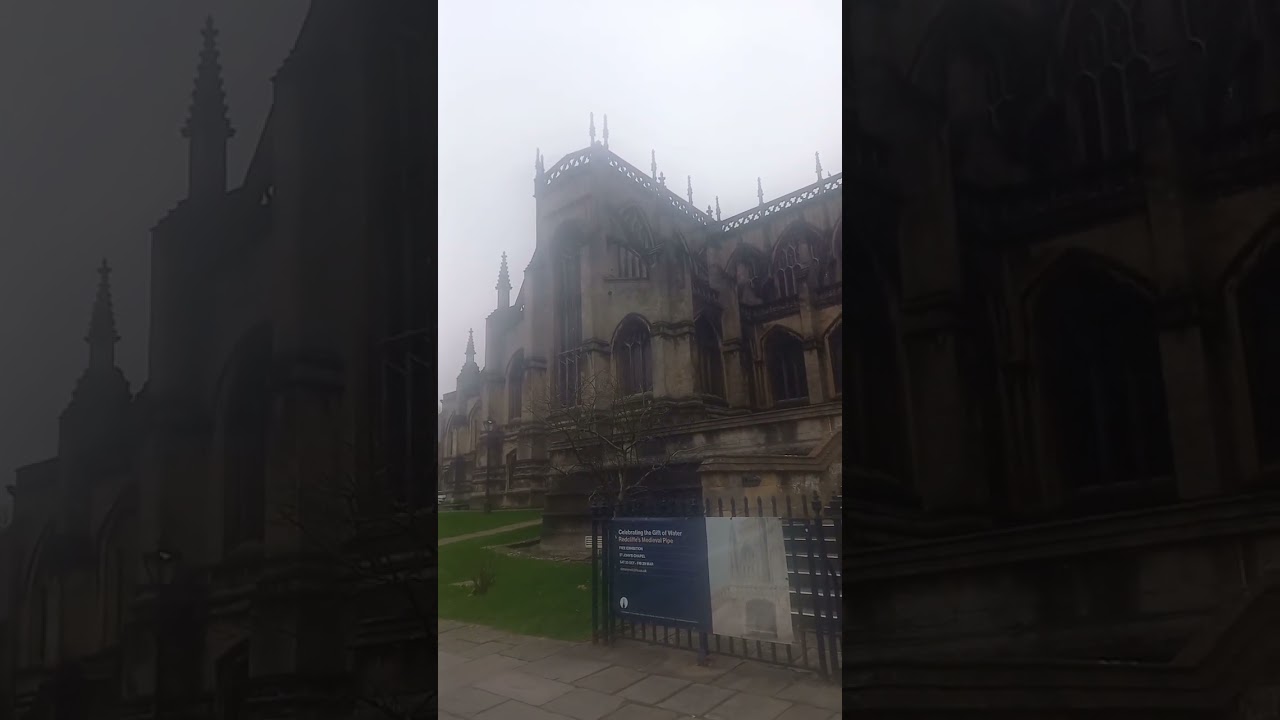The photograph features a grand, round, beige stone building that appears to be a cathedral or museum with multiple steeples and barred windows. The image is divided into three parts, creating a panoramic effect. The central section is well-lit, showcasing the building in daylight, revealing a green lawn and a stone cobblestone sidewalk leading up to its entrance. There is an iron fence in front of the building displaying a banner, which partially reads "celebrating the gift of," though the rest of the text is too small to decipher. The left and right sections of the photograph are artistically darkened and obscured, showing only the faint outlines and edges of the structure, with the right section providing a closer view of the windows.